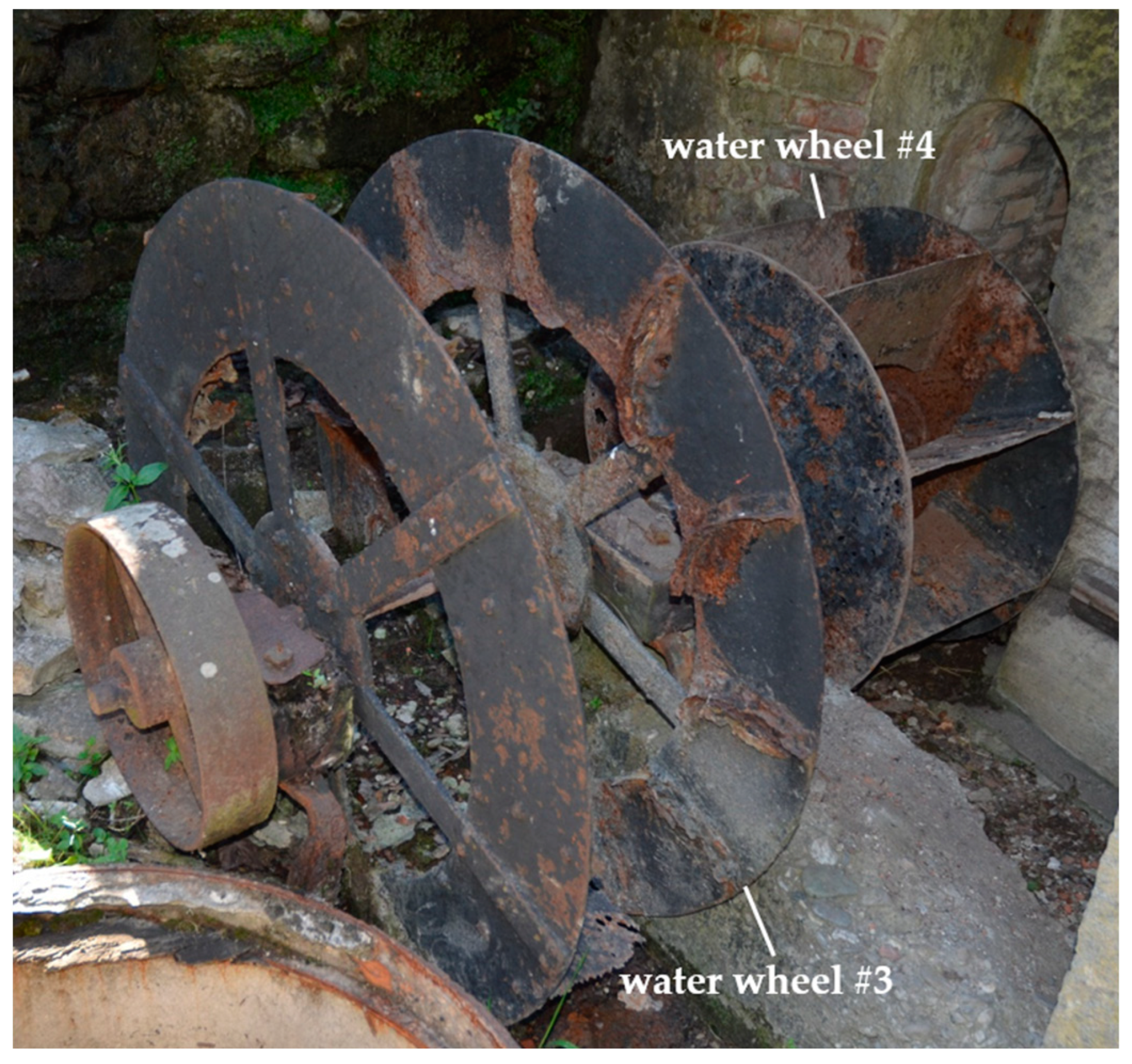This is a detailed real-life photograph taken from above, showcasing two ancient, highly rusted water wheels, presumably from a grist mill or water mill. Both water wheels are covered in red corrosion and situated outdoors on a base of broken gray rocks, suggesting they haven't been moved since their last use. The photograph includes white labels identifying the wheels: "water wheel number four" and "water wheel number three," with respective lines pointing to each.

Water wheel number three, which occupies the left half of the image, features two large, flat disks with holes at their centers, connected by an axle and round bolts, indicating structural details. The right side of the image holds water wheel number four, which consists of two solid disks joined by paddles between them, designed to carry water as the wheel turns.

The setting includes elements like a rusted pot fragment in the bottom left corner and small green weeds sprouting among the rocks, adding to the abandoned and decayed atmosphere. Dominant colors in the photograph are the grays of the metal and rocks, contrasted with the orange hue of rust, highlighting the extensive corrosion and historical wear of these industrial relics.